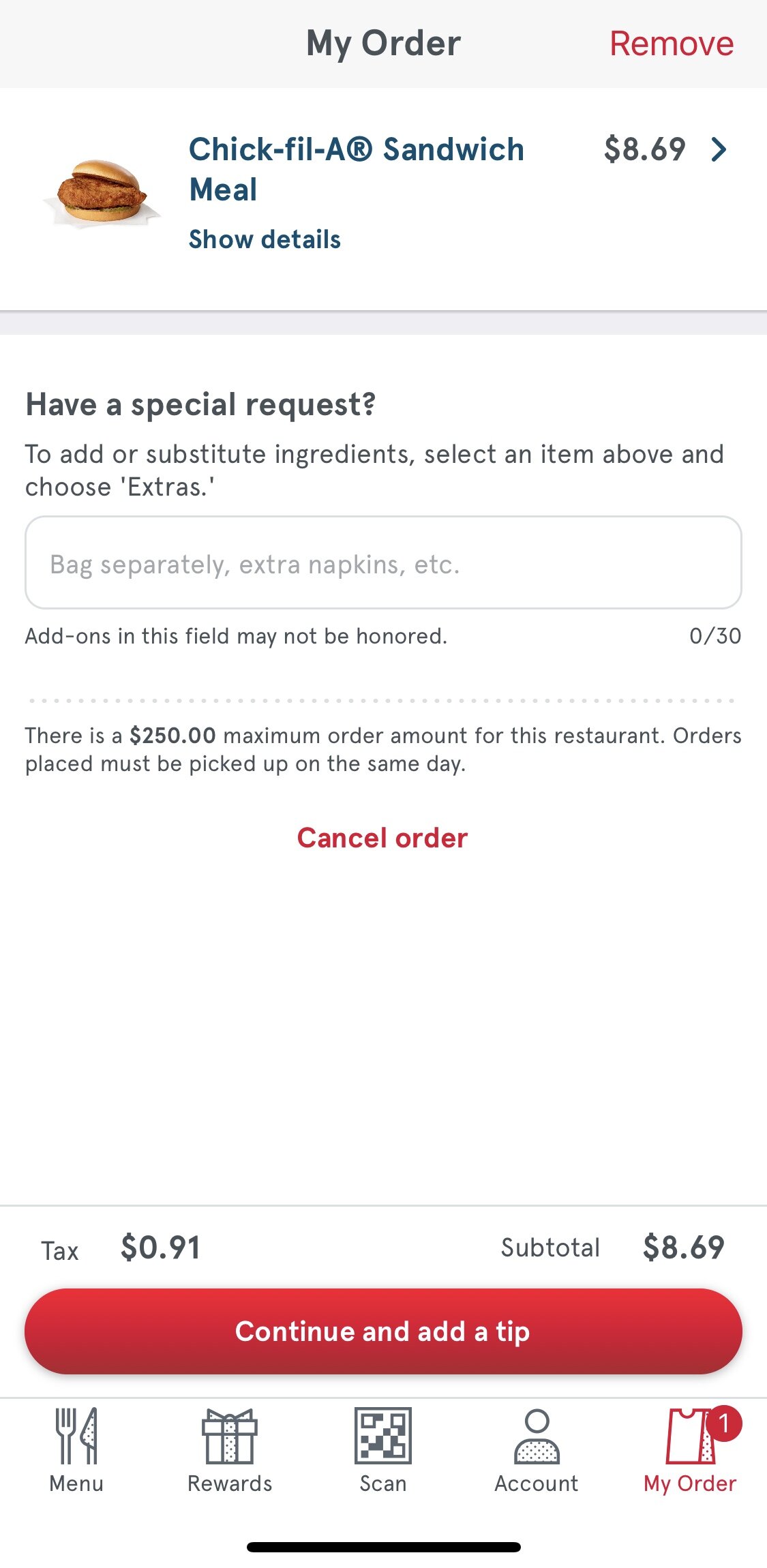Screenshot of a Chick-fil-A Mobile App Order Summary:

At the top of the screenshot is a gray bar featuring the text "My Order" centered, with the option "Remove" in red on the right end of the bar. Directly below this, there is a white section displaying an image of a Chick-fil-A sandwich to the left. This section is labeled "Chick-fil-A Sandwich Meal" with the option to "Show Details" written underneath the label. On the far right of this section, the price is listed as $8.69 accompanied by a right-facing arrow.

Following this, a separator bar leads into a white background blurb that reads: "Have a special request to add or substitute ingredients? Select an item above and choose extras." Below this blurb is an open text field placeholder reading "Bag separately, extra napkins, etc." in grayed-out text. A note beneath this field states, "Add-ons in this field may not be honored." On the far right of this section, there is a character limit indicator showing "0/30."

Below the dotted separation line, there is an informational note stating, "There is a $250 maximum order amount for this restaurant. Orders placed must be picked up on the same day."

Toward the bottom of the screenshot, a red "Cancel Order" button is prominently displayed. A substantial space follows, leading to another line break with the tax amount of $0.91 listed on the left and a subtotal of $8.69 on the right. Below this, there is a prominent red button labeled "Continue and Add Tip."

At the very bottom of the screenshot is the navigation bar, which includes icons labeled from left to right: Menu, Rewards, Scan, Account, and My Order.